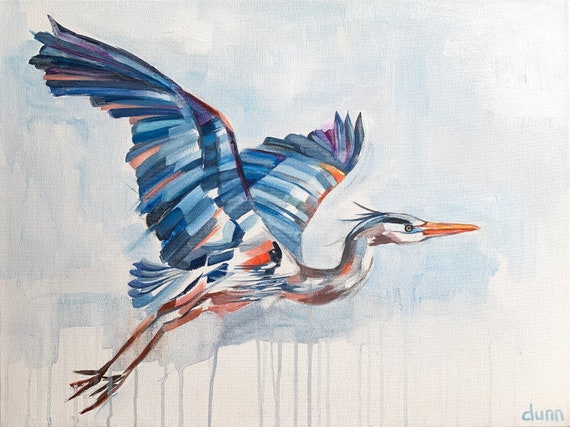This detailed description combines and enhances the elements from each voice caption:

This is a watercolor painting of an egret in flight, positioned centrally and moving towards the right side of the image. The egret's wings are gracefully outstretched, displaying a stunning array of shades, including light and dark blues, touches of black, a bit of purple, and hints of orange. The bird's body features a harmonious blend of orange, various blues, muted reds, and peach tones. The egret's longer neck transitions to a head adorned in shades of gray, blue, and white, accented with an orange beak and a distinct black line above the eyes. The slender legs are painted in peachy tan hues, hanging down with visible claws.

The background of the painting enhances the bird's vibrant colors with subtle washes of light blue and gray, exhibiting the characteristic drip effect typical of watercolor art. In the lower right-hand corner, the painting is signed by the artist in light blue letters, reading "DUNN." This detailed rendering vividly captures the elegance and motion of the egret, showcasing the artist's skill in watercolor technique.